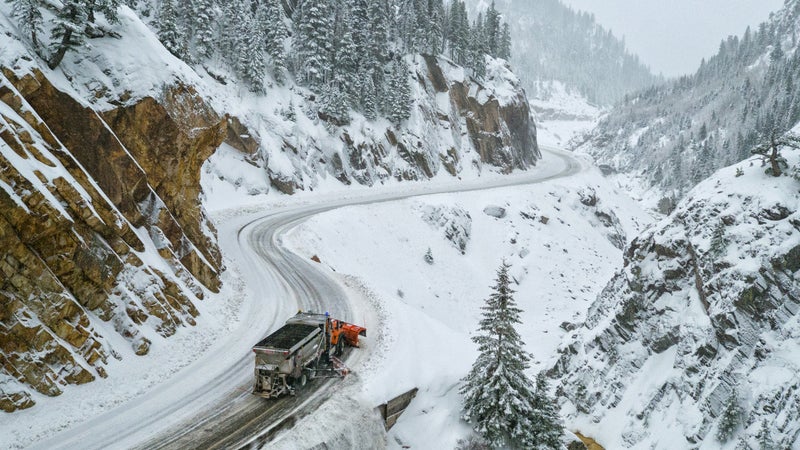This horizontally aligned rectangular image captures a stunning winter scene taken from atop a hill, looking down onto a snowy mountain road. On the left side stretching to the middle of the photograph, a steep cliffside of mostly brown rock transitions to being heavily covered in snow, interspersed with snow-laden pine trees. Moving towards the right, the upper part of the image reveals a gray, cloudy sky contrasting with the snowy landscape below. In the foreground on the right, another large rocky cliff appears, this one almost entirely blanketed in snow with a prominent pine tree jutting out from the bottom and middle. Below it, near the cliff’s base, a truck equipped for snow shoveling can be seen driving along a curved, well-traveled road that runs from the bottom left into the middle, eventually disappearing into the background. The road, bordered by banks of snow, shows a thin layer of snow, indicating frequent use. The truck has an orange and silver (or green) body with a red bumper, diligently making its way through the frosty terrain amidst the blurred outline of distant, snow-covered mountains and trees, under the expansive, cloudy sky.